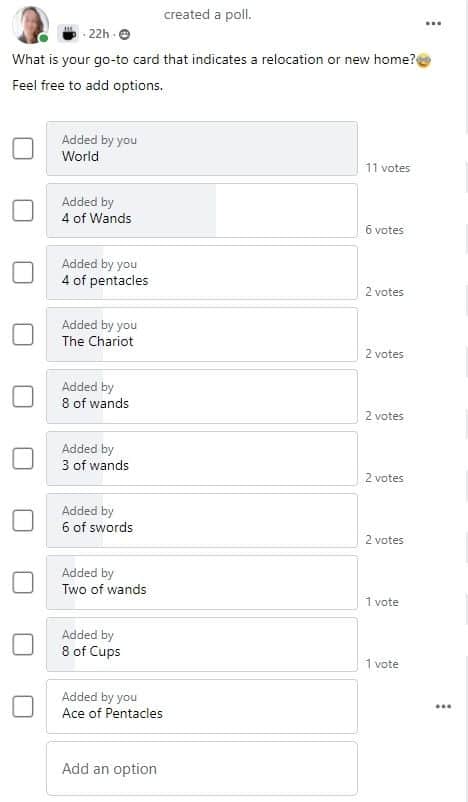The image depicts a social media post, likely on Facebook, featuring a poll about finding resources for relocating to a new home. The top section presents a profile of a woman with shoulder-length brown hair and a light skin complexion, wearing a dark green shirt. A small green circle beside her picture indicates she is online.

Next to her image is a dark grey square icon with a black coffee cup emitting small steam lines. To the right, text in grey reads "22 hours ago" next to a white silhouette of multiple people.

The poll question, written in black text, asks: "What is your go-to card for indicating a relocation to a new home?" This text is followed by an emoji with glasses and instructions saying "Feel free to add options."

The responses include various tarot card names along with their vote counts:
1. "Added to you world" with 11 votes.
2. "Added by 4 of wands" with 6 votes.
3. "Added by you 4 of pentacles" with 2 votes.
4. "Added by you The Chariot" with 2 votes.
5. "Added by 8 of wands" with 2 votes.
6. "Added by 3 of wands" with 2 votes.
7. "Added by 6 of swords" with 2 votes.
8. "Added by 2 of wands" with 1 vote.
9. "Added by 8 of cups" with 1 vote.
10. "Added by you Ace of Pentacles."

At the bottom, there is an option to add more responses, and the left-hand side displays squares without check marks.